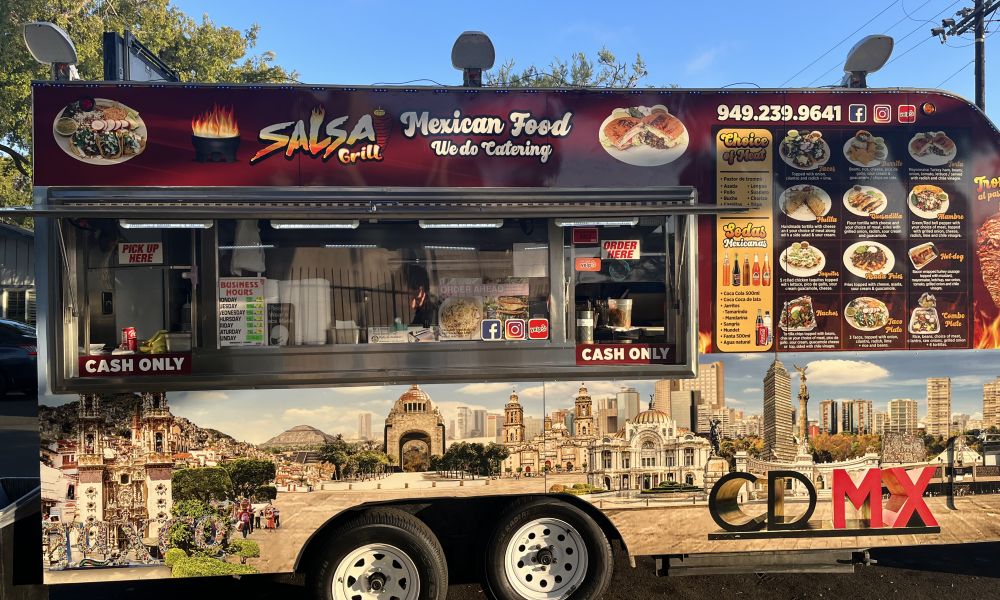This close-up photo showcases the intricately detailed side of a maroon food truck titled "The Salsa Grill." The scene is set against a backdrop featuring a couple of Chinese characters, a power pole, power lines, and a clear blue sky. The exterior of the food truck is adorned with vibrant photos of their menu items and a mural wrap of a Mexican town, marked with 'CDMX' in the lower right corner. The truck’s open serving window is flanked by clear signs: "Order Here" on the right and "Pick Up Here" on the left, both indicating "Cash Only" on either side. Additionally, the window displays the business hours. The menu, located at the top right of the truck, includes various food and drink options and is accompanied by a phone number and logos for Facebook, Instagram, and a food delivery service. The truck proudly advertises "We Do Catering." The reflection of gates opposite the truck is visible in the window, adding to the dynamic composition of the photograph.